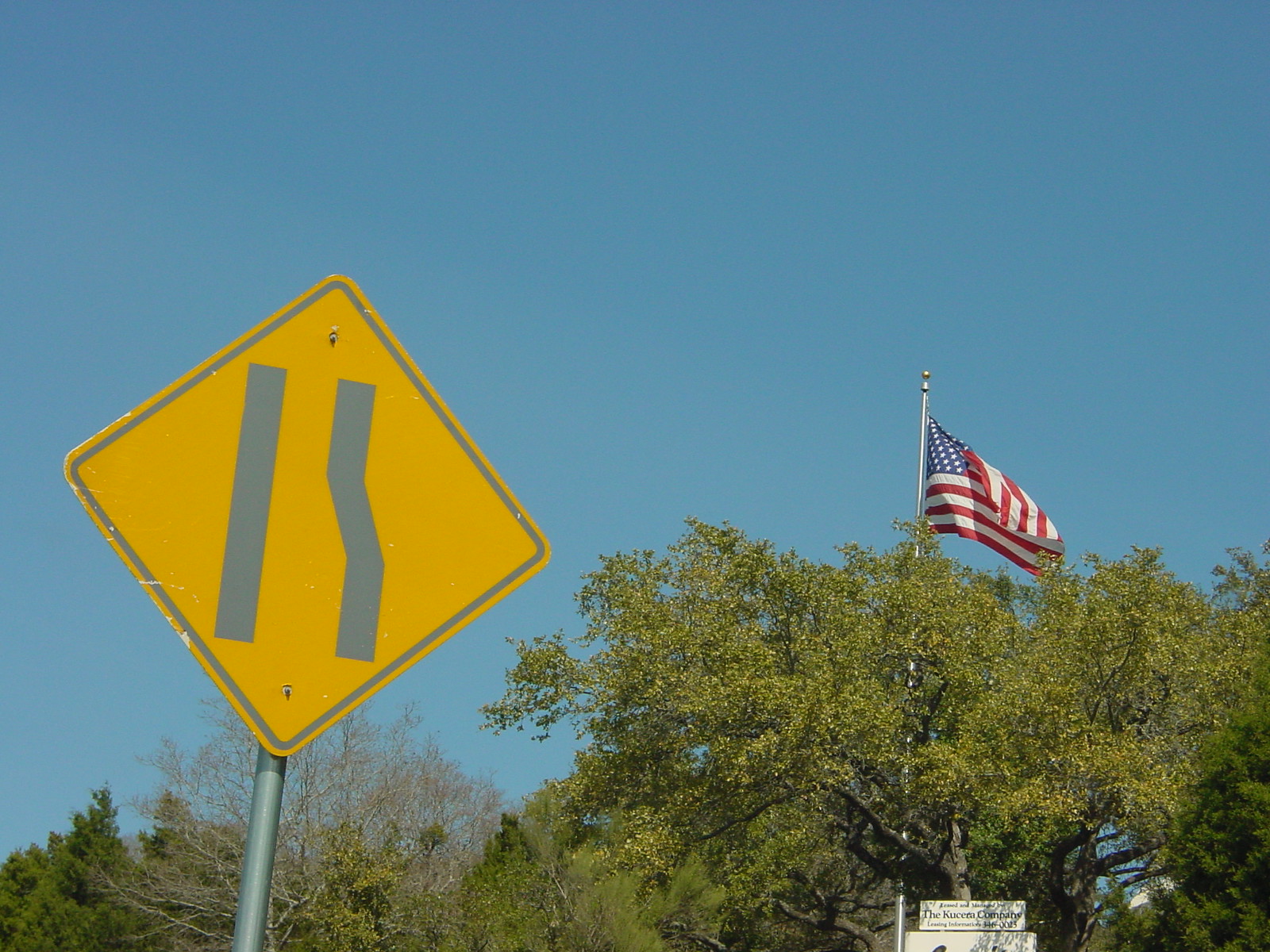The image captures a yellow, diamond-shaped road merging sign prominently displayed in the center. The sign features two lines, one straight and the other curving, indicating a merging lane ahead. This sign is situated on a silver pole and bordered with a light gray edge. The background presents a vivid, clear blue sky occupying the upper portion of the image, extending down to about two-thirds of the frame. Below the sky, a tree line begins roughly two inches from the bottom of the image, with various trees scattered across.

To the right of the sign, there is a distinctly lush, green tree, whose dense foliage stretches upward covering a part of the scene. Embedded within the treetops, about two inches from the right edge of the image, an American flag is visible, fluttering in the breeze on a silver pole, partially obscured by the surrounding vegetation. A barren tree branch, located closer to the camera and directly behind the sign, extends into the shot, adding contrast to the otherwise verdant scenery. Additional green trees also populate the left side of the image, complementing the serene, mid-day atmosphere.